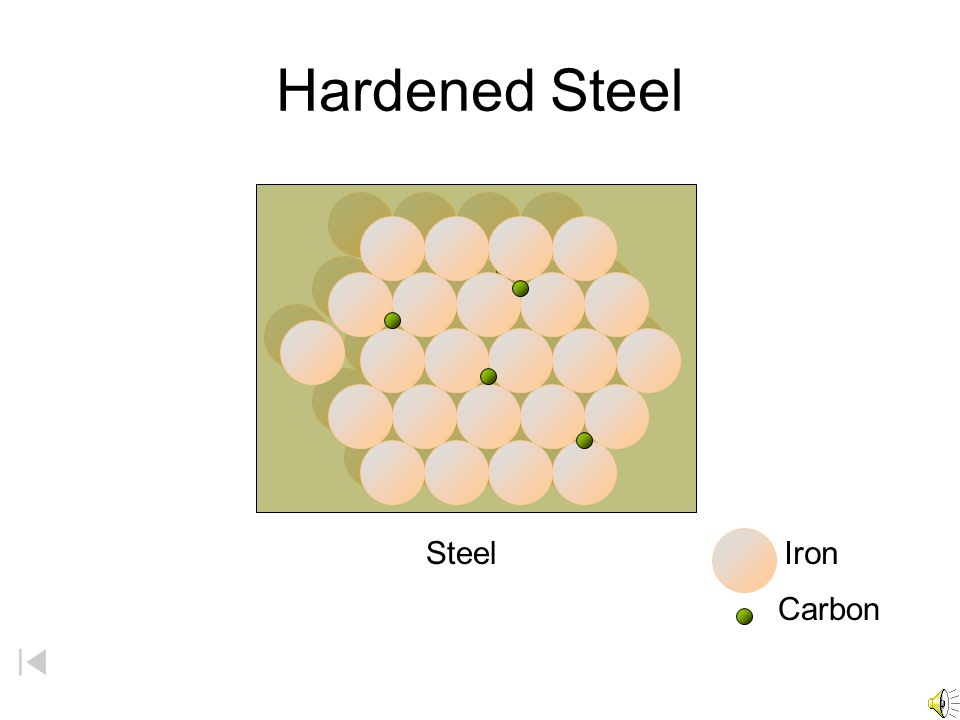The PowerPoint slide titled "Hardened Steel" features a detailed image illustrating the composition of steel. The slide has a white background with black text, and the image itself showcases a light olive green backdrop adorned with numerous large pink circles representing iron atoms. Scattered among these pink circles are smaller green dots signifying carbon atoms. The image is labeled "steel" beneath the depiction. In the bottom right corner, a legend clarifies the color coding: pink circles for iron and green dots for carbon. Additionally, there are navigation symbols, with an audio symbol in the very bottom right and a back arrow in the bottom left, ensuring user-friendliness. The meticulous arrangement within the image visually communicates the molecular structure of hardened steel, highlighting the predominance of iron (with more than 20 pink circles) and a sparse distribution of carbon (only four green dots).